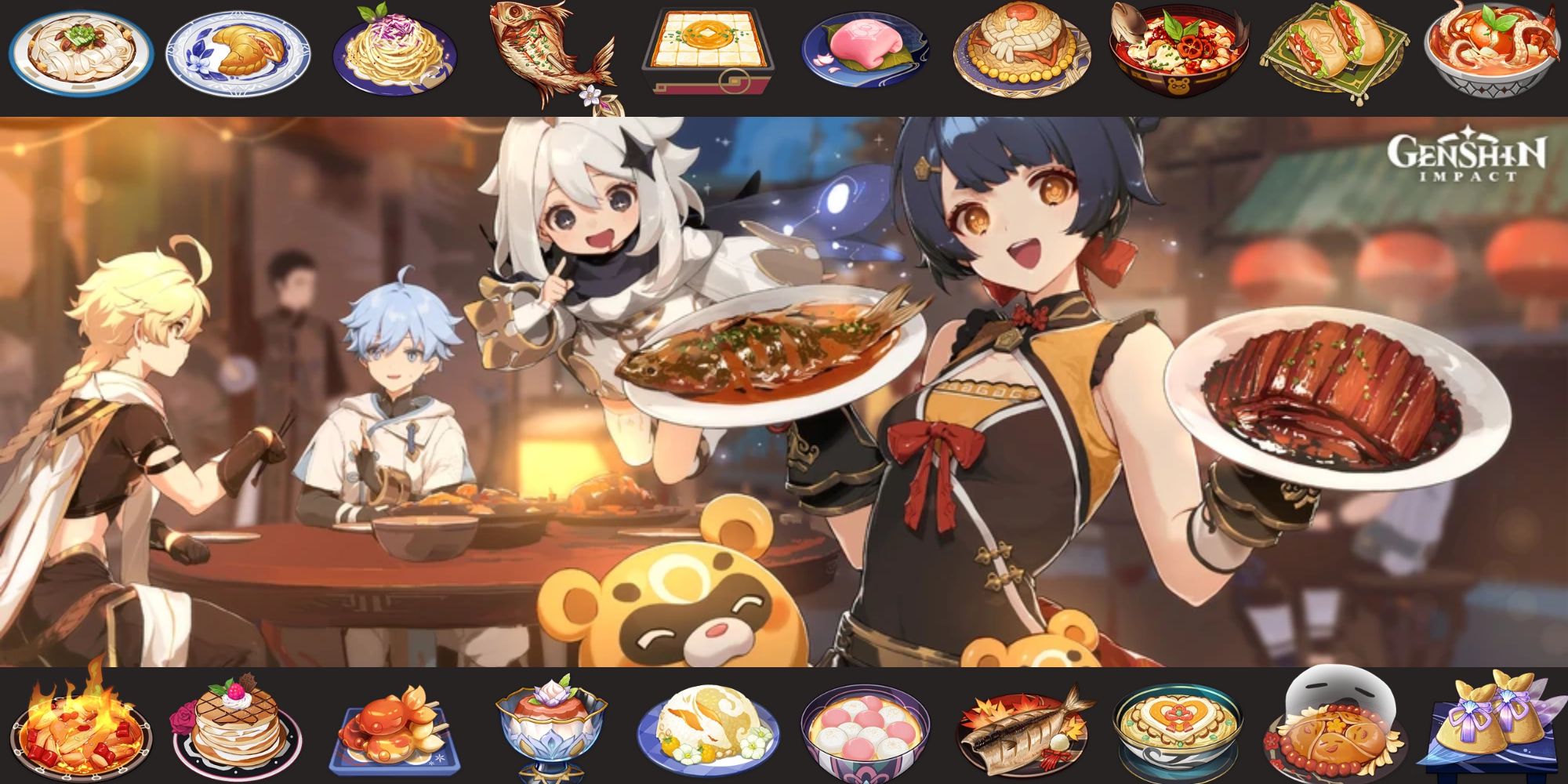This is a detailed screenshot from the anime-style game Genshin Impact, featuring a richly depicted scene. The image prominently displays an anime girl with short black hair and large expressive eyes standing in the foreground. She is dressed in a chocolate brown and tan costume, holding a large plate of braised fish in one hand and another dish resembling pork belly in the other, tipping them towards the viewer for a closer look. Below her, there's an adorable anime-style teddy bear with chocolate markings around its eyes, giving a playful touch to the scene. The background reveals a cozy, inviting atmosphere with two other anime characters—one with blonde hair and the other with blue hair—seated at a wooden table, possibly engaged in a conversation. A warmly lit fireplace adds to the setting's charm. The top and bottom of the image are framed by black borders adorned with various food depictions, ranging from noodle dishes and fish to bowls of stew and delectable desserts, suggesting options that can be made or encountered in the game. The Genshin Impact logo is elegantly displayed in white on the upper right corner, enhancing the promotional aspect of the image.